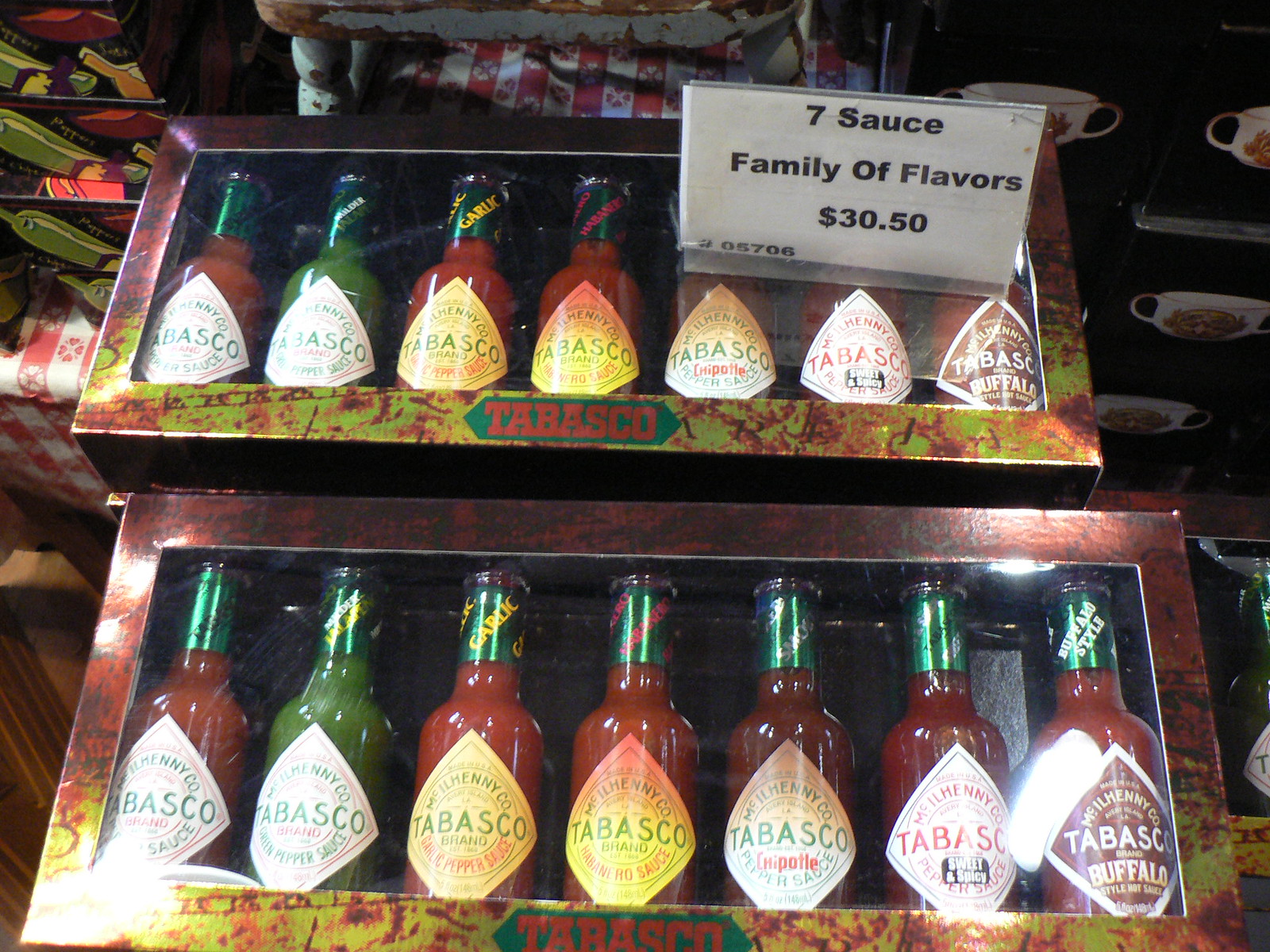This color photograph, likely taken inside a store, captures a close-up view of two gift boxes of assorted Tabasco sauces prominently filling the frame. Each box contains seven different bottles of Tabasco sauce, featuring flavors such as Buffalo, Sweet & Spicy, Chipotle, Habanero, Garlic Pepper, Chili Pepper, and the classic regular Tabasco sauce. The sauces are packaged in a copper, orange, and yellow-colored box with a clear window at the front, showcasing the vibrant labels and varying hues of the sauces inside—ranging from green to various shades of red. A white sign with black type displayed above the boxes reads, "Seven Sauce, Family of Flavors, $30.50," with the number 05706 noted in the lower left corner of the sign. The background includes a gingham tablecloth, the back of a chair, and several double-handled soup bowls or cups, adding context to the store setting. The photograph is taken in landscape format, emphasizing the detailed and organized presentation of the products.